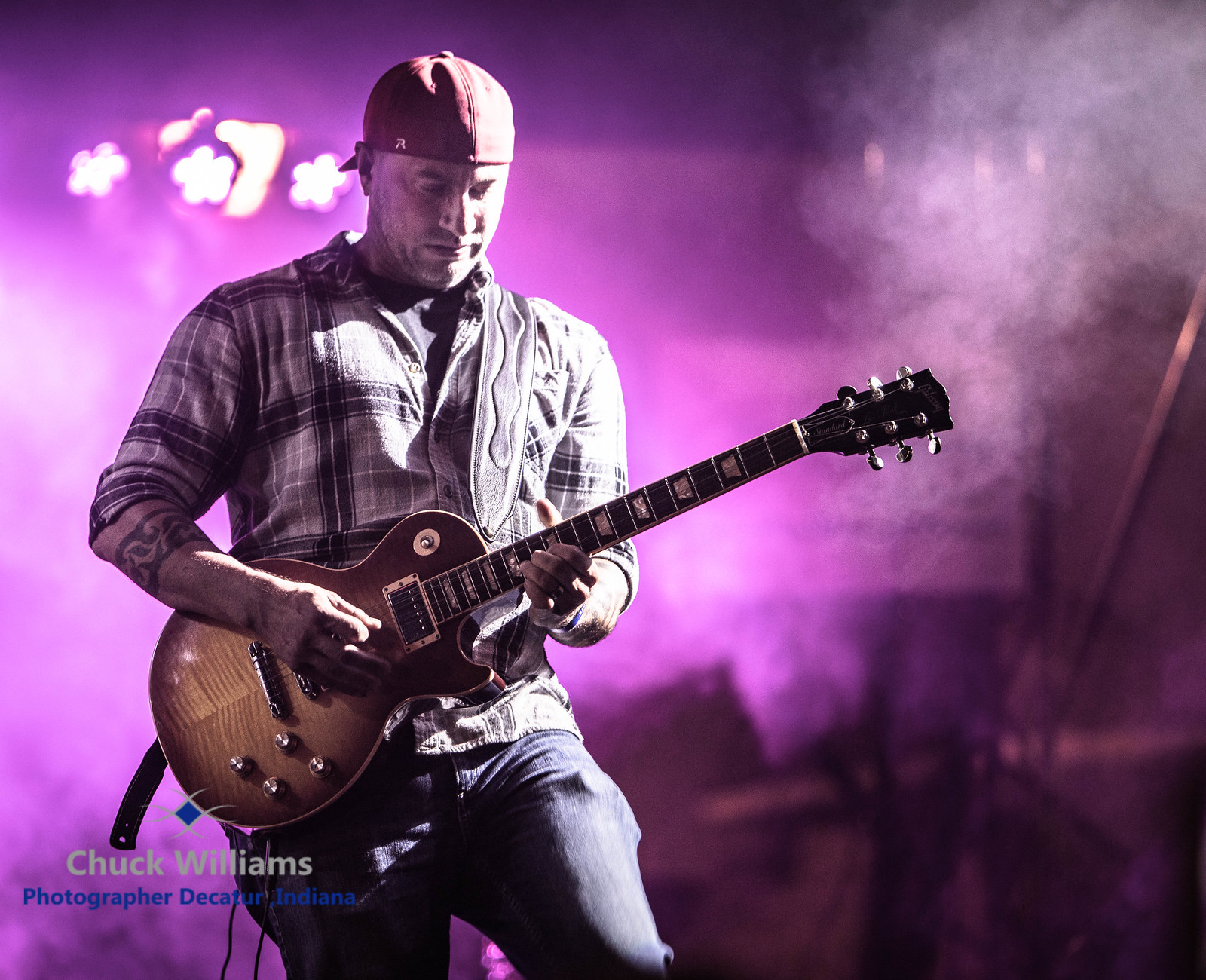In this image, we see a man at the center of a dimly lit indoor concert, captured mid-performance. He's wearing a black and white flannel shirt with sleeves rolled up, a red backwards hat, and jeans. The man is playing an electric guitar that has a distinct, stylish look similar to an acoustic guitar, with bright, vivid colors. The background features concert equipment and is lit with a variety of colors including purple, pink, blue, orange, and shades of gray, giving a vibrant yet smoky ambiance. A text watermark at the bottom of the image reads "Chuck Williams, photographer, Decatur, Indiana," accompanied by a logo above it in gray and blue. This visually striking photograph, with dramatic lighting and a touch of performance smoke, captures the essence of a live music event.